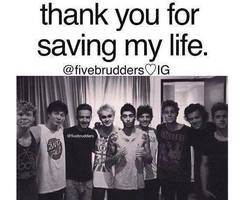The small, black and white photograph captures a group of seven young men standing shoulder to shoulder, posing confidently. Their ages appear to range from teenagers to young adults. Each individual sports different attire, including t-shirts, some with band logos, and the central figure wearing a sleeveless tank top, showcasing arm tattoos. The men are of similar height and positioned in what seems like a room with an open door in the background and a curtain hanging behind them. The scene is intimate and evokes a sense of camaraderie. Above the image, text in black on a white background reads, "Thank you for saving my life," attributed to "5BrothersHeartIG." This appears to be a heartfelt tribute or expression of gratitude.